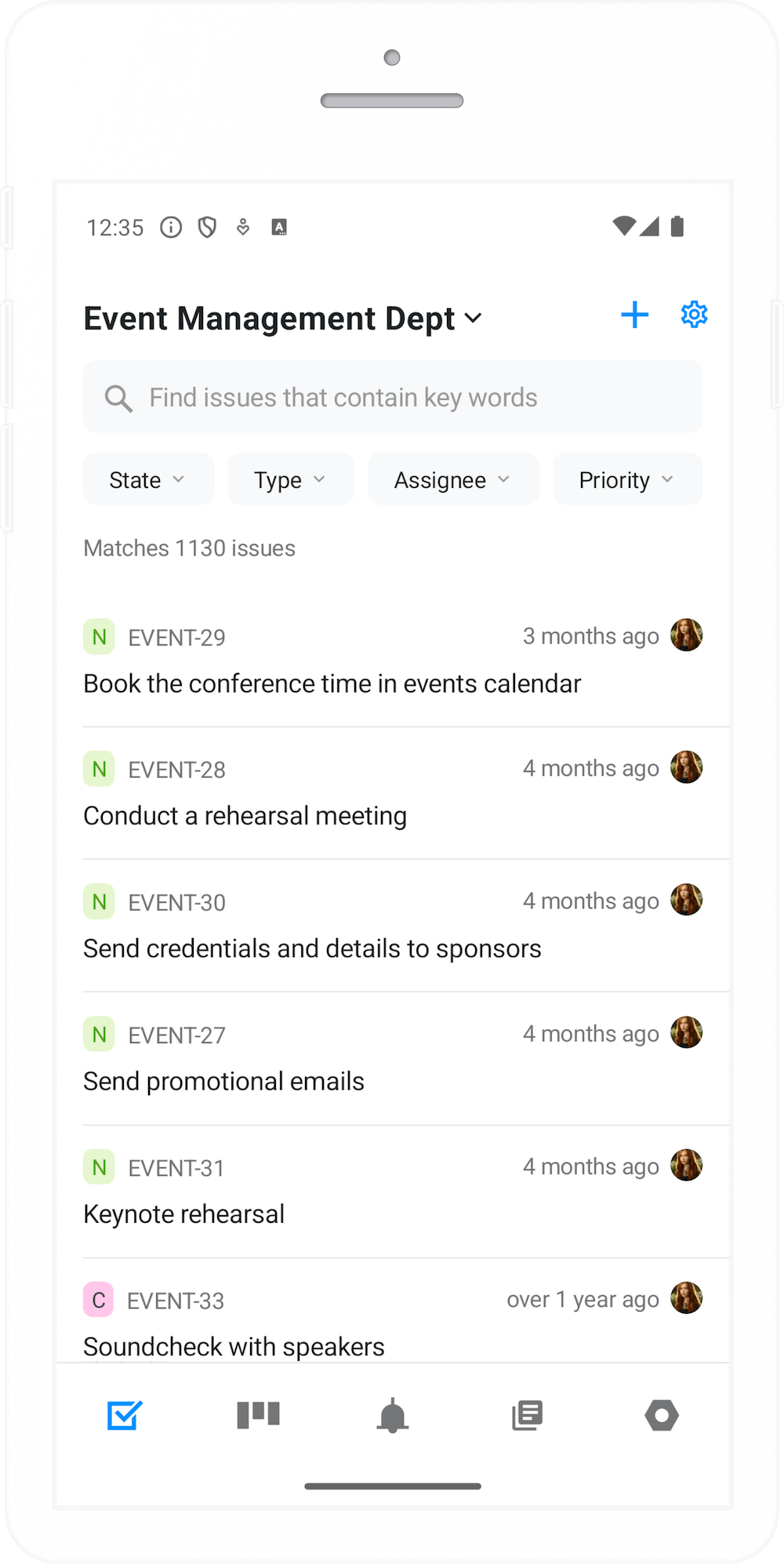This is a detailed screenshot of an Android phone's interface, not an iOS device. At the top of the screen, the time is displayed as 12:35. To the right of the time are several icons: an information icon represented by an eye, a shield icon, a profile image, the letter "A," and icons for Wi-Fi, cellular signal, and battery status, all indicating full capacity—100% battery, full Wi-Fi signal (3 out of 3 bars), and full cellular signal (4 out of 4 bars).

Beneath this, the title "Event Management Department" is prominently displayed with a drop-down arrow to its right. Adjacent to the title are a blue plus sign and a blue settings icon. Below this title bar is a search bar with the placeholder text "Find issues that contain keywords," accompanied by four subcategory filters: State, Type, Assignee, and Priority.

A small text below the search bar indicates "Matches 1,130 issues." Listed below are several items, each following a consistent format:

1. **End Event 29** - 3 months ago: "Book the conference time and events calendar."
2. **End Event 28** - 4 months ago: "Conduct a rehearsal hearing."
3. **End Event 30** - 4 months ago: "Send credentials and details to sponsors."
4. **End Event 27** - 4 months ago: "Send promotional emails."
5. **End Event 31** - 4 months ago: "Keynote rehearsal."
6. **C Event 33** - Over 1 year ago: "Soundcheck speakers."

Noteworthy is that all "N" indicators appear in green, while the "C" indicator is in pink.

At the bottom of the screen, five icons indicate the current section, providing additional navigation options within the application.